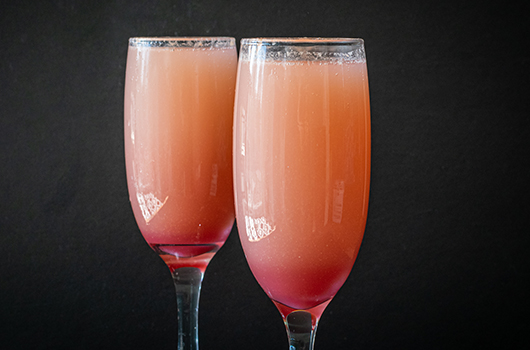In this photograph taken indoors, two long-style cocktail glasses are prominently featured at the center. Positioned slightly offset, with the glass on the left slightly behind the one on the right, both are filled nearly to the brim with a vibrant orange-pink liquid, likely a grapefruit or peach-based cocktail. The glasses stand against a stark black background, emphasizing their contents. Light reflections from a window and what appears to be a white stove create illuminating patterns on the glasses' surfaces, particularly noticeable at their bases. The liquid inside transitions subtly from a gentler pinkish hue at the bottom to a richer cream-orange color near the top. Both glasses are mounted on elegant glass stems and remain untouched, filled to their intended levels, suggesting they are ready to be enjoyed. The dark background ensures the glasses and their colorful contents remain the focal point of the image.